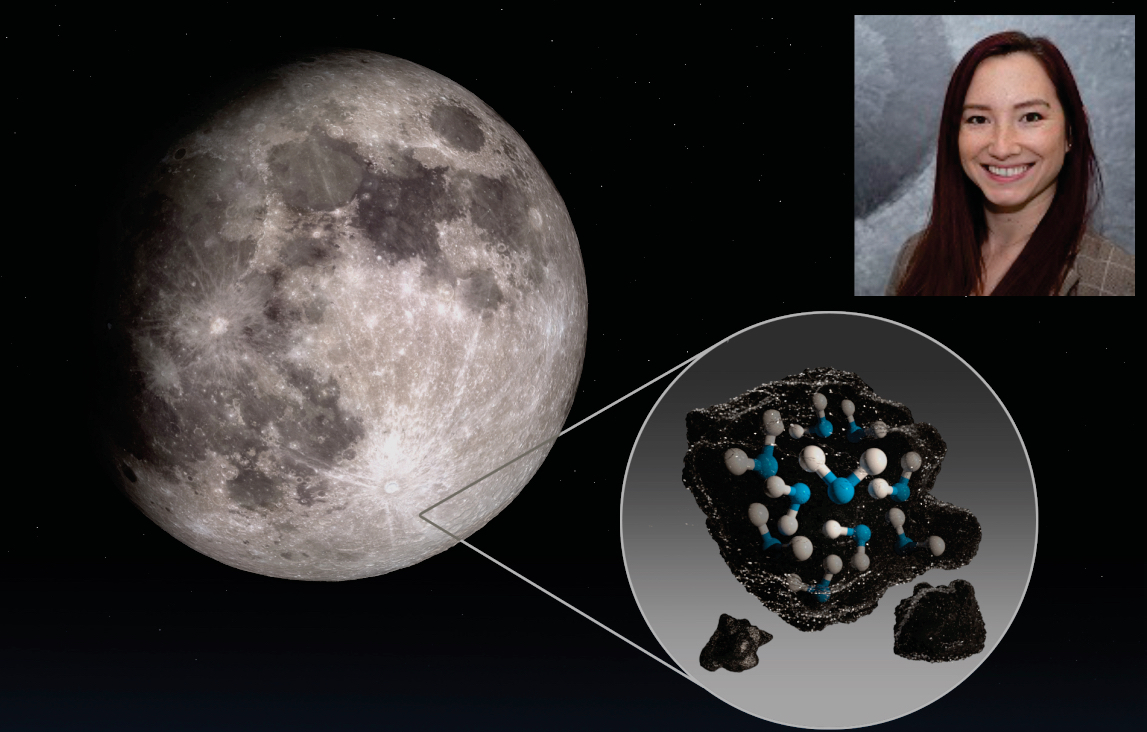The image is a horizontally aligned rectangular picture with a solid black background. Dominating the left side is a realistic depiction of the moon, shown in shades of gray with dark spots. The far left edge of the moon blends into the black background. From the lower portion of the moon, two diagonal lines extend, forming a sideways V shape. These lines point towards a zoomed-in circular inset detailed with a white outline. Within this circle, there are blue and white molecules set against a black, rock-like textured background. The inset appears to illustrate the composition of the moon's surface. In the upper right corner, there's a small square image of a smiling white woman with long dark hair, parted in the middle. She's wearing a brown plaid jacket and possibly a gray and white blouse underneath. This woman may be related to the discovery depicted in the illustration.